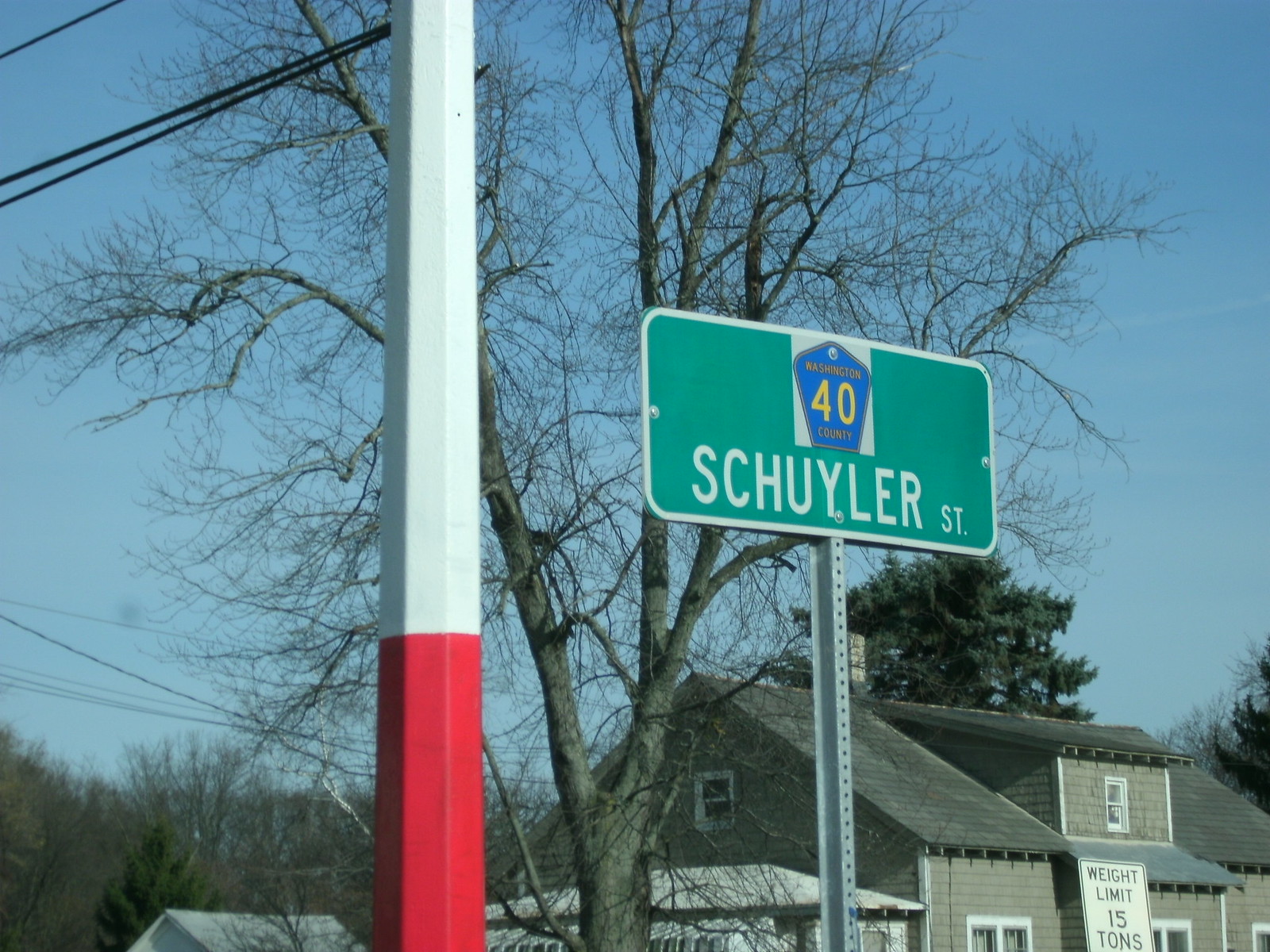In this vibrant color photograph, a tall pole, predominantly white with a red base, stands prominently near the center but slightly to the left. Affixed to the pole is a green street sign that reads "Schuyler Street" in white letters, accompanied by a blue shield emblem that designates "Washington County 40" in yellow text. A smaller sign, positioned to the right, indicates a weight limit of 15 tons. The backdrop features a charming two-story brown clapboard house, partially obscured by a large tree situated between the pole and the green sign. Additional trees, rich with foliage, fill the background, while telephone wires trace a path across the top-left corner and lower-left edge of the image. The scene is bathed in clear, bright sunlight, with a flawless blue sky overhead, completing the picturesque setting.